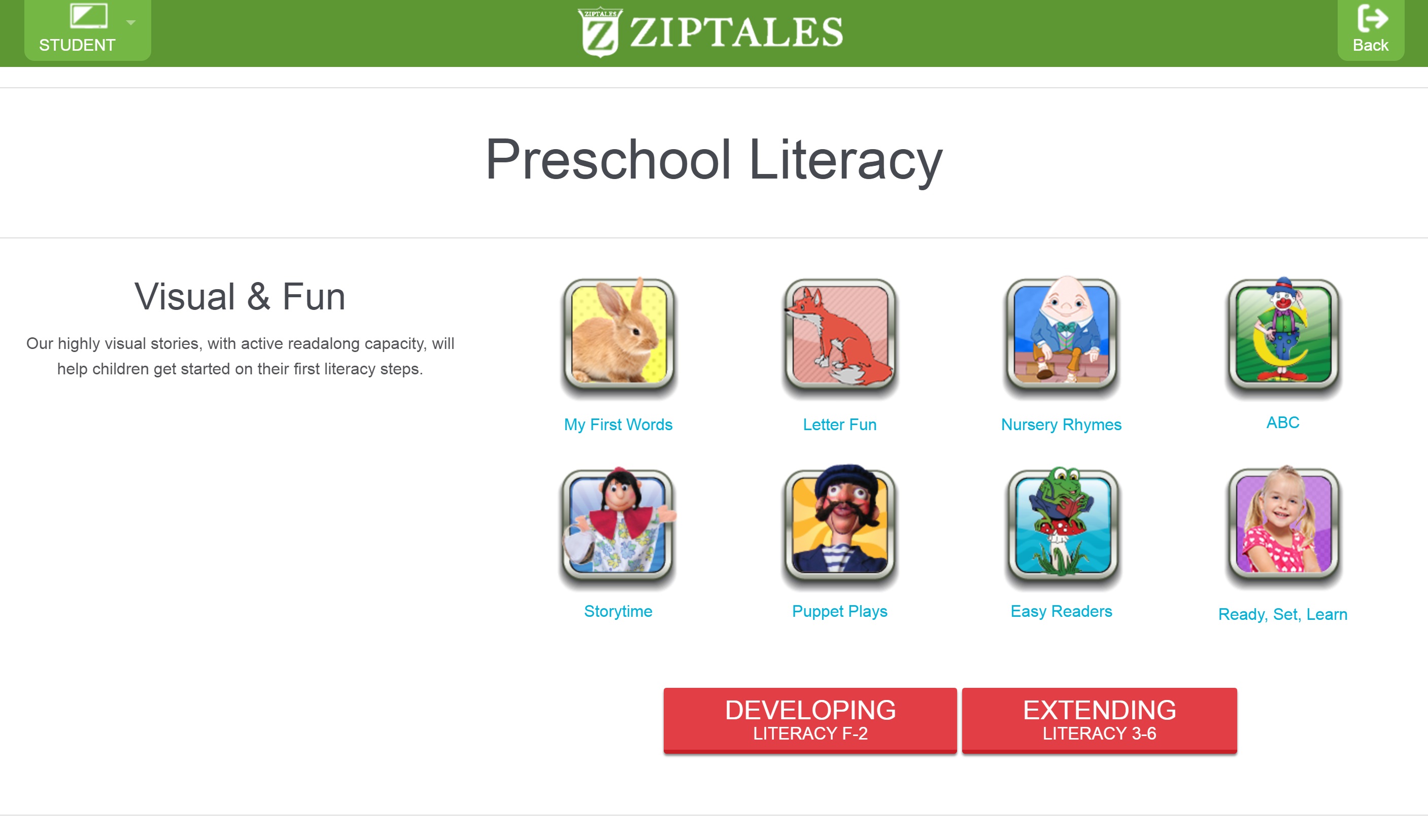The homepage of a preschool learning website titled "ZipTales" is prominently displayed, with the title centrally positioned at the top in bold white font. To the left of the title, the site's logo is visible, featuring a shield with a bold "Z" in the middle. On the top left corner of the screen, there's a drop-down menu button labeled "Student," accompanied by an icon resembling a rectangular device, possibly a computer screen, with a white triangle in the upper left corner. On the top right, there is a back button symbolized by a small door with an arrow pointing outwards. The main content of the webpage highlights "Preschool Literacy," followed by the phrase "Visual and Fun." Below this, the site explains its mission, stating: "Our highly visual stories with active read-along capacity will help children get started on their first literacy steps."